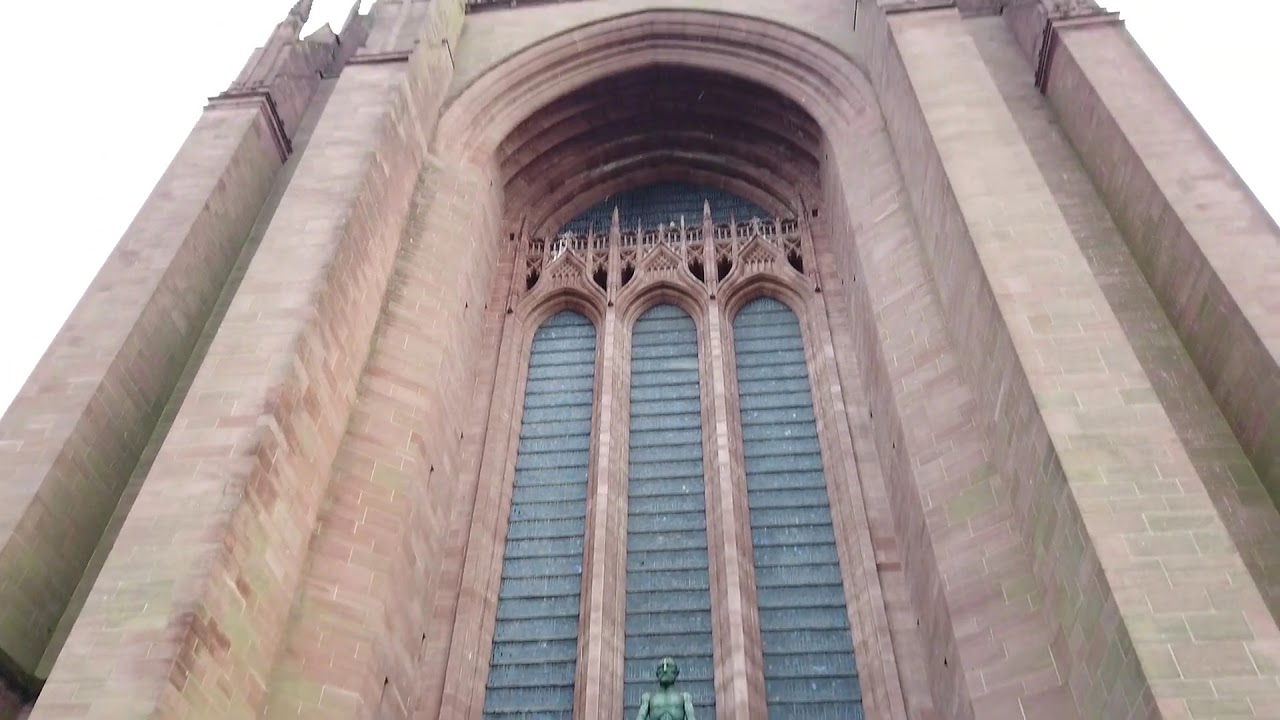The image captures a detailed, upwards perspective of a Gothic-style building, emphasizing its vertical grandeur. The gray cemented structure, adorned with pointed tops and ornate designs, features a large, curved, arched window in the center with multiple rectangular frames and intricate spikes at the top. The window is flanked by columns exhibiting light blue stripes, adding a touch of color to the otherwise monochromatic palette. At the bottom center of the shot, a grayish-green statue of a person or religious figure stands prominently. The building's walls exhibit varying shades of red and pink, enhancing the visual depth and historic appeal. Captured from the base looking up, the photograph accentuates the building's timeless and towering architecture.